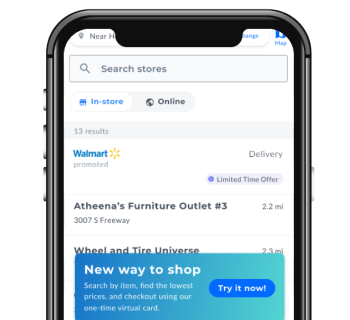The image showcases the top half of an iPhone screen displaying the Walmart app. The very top of the screen is partially obscured, but the visible part clearly indicates the 'Search stores' function with options for 'In-store' and 'Online' shopping. The search yields 13 results.

The first result appears to be a Walmart promotion for their delivery service, noting a 'Limited Time Offer.' Following this, the second result is for 'Athena's Furniture Outlet', listed as 2.2 miles away, with the address of 3007 S Freeway. The third result, 'Wheel Entire Universe,' shown to be 2.3 miles away, is partially covered by a pop-up message.

The pop-up message reads: "New way to shop: Search by item, find the lowest prices, and check out using our one-time virtual card." Adjacent to this message, there is a blue button with white text that says "Try it now."

Overall, the iPhone is set against a stark white background, providing a crisp and clean context for the displayed information.